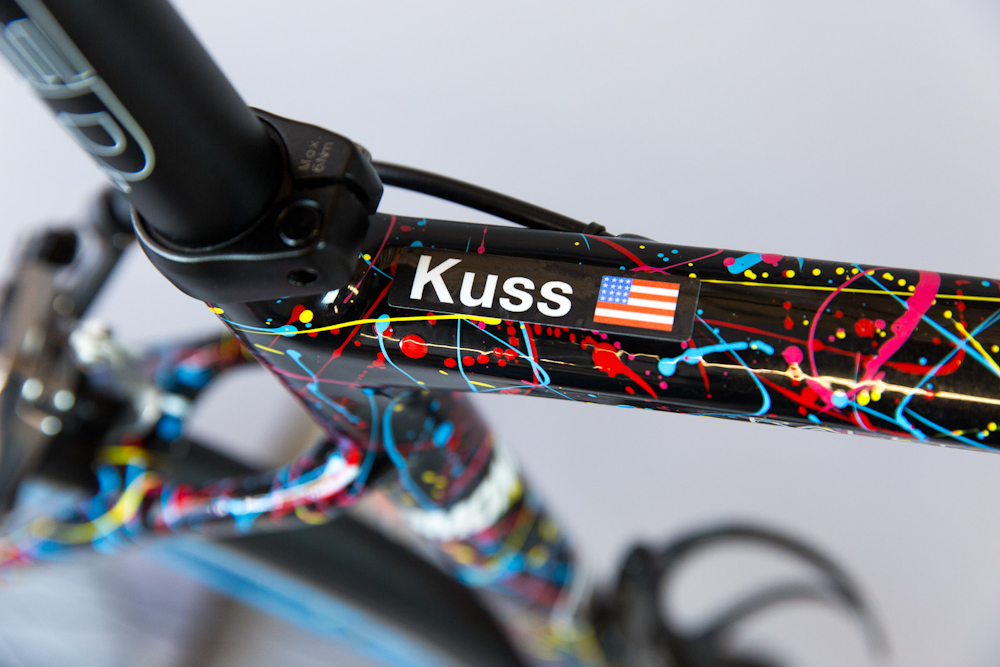The image is a close-up of a black bicycle, specifically focusing on its crossbar and part of the handlebar setup. The crossbar prominently features a label that reads "KUSS," spelled out as K-U-S-S, accompanied by an American flag decal. The black background of the bicycle's frame is adorned with vibrant, multicolored paint splatters, including shades of blue, pink, yellow, and red, creating an abstract design. The left side of the image reveals a partially visible tire with a light blue inner lining and the brake mechanism, including the cord extending towards the handlebar. The lower half of the image is blurry, emphasizing the sharp focus on the crossbar and the adjacent black frame leading up to the handlebars. The background of the photo is a light gray, contrasting with the dark, shiny steel of the bicycle.